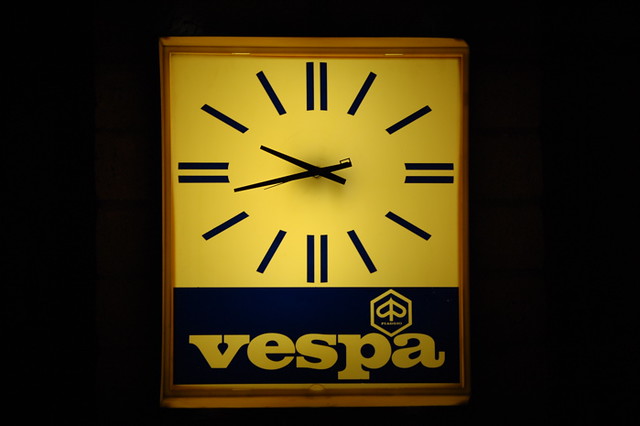A striking image features a classic clock set against a pristine black background. The clock, centered perfectly within the frame, draws immediate attention with its distinctive and minimalistic design. Sporting numerals "1" and "2" instead of the conventional full set of numbers or Roman numerals, the clock's face emanates a warm, yellowish hue. The black hour and minute hands stand out sharply against the face, ensuring easy readability. At the bottom of the dial, the logo "VESPA" is prominently displayed in elegant black lettering, though it is unclear whether this is related to the renowned scooter brand or represents a different entity. The simplicity and elegance of the clock's design make it an aesthetically pleasing focal point in the image.